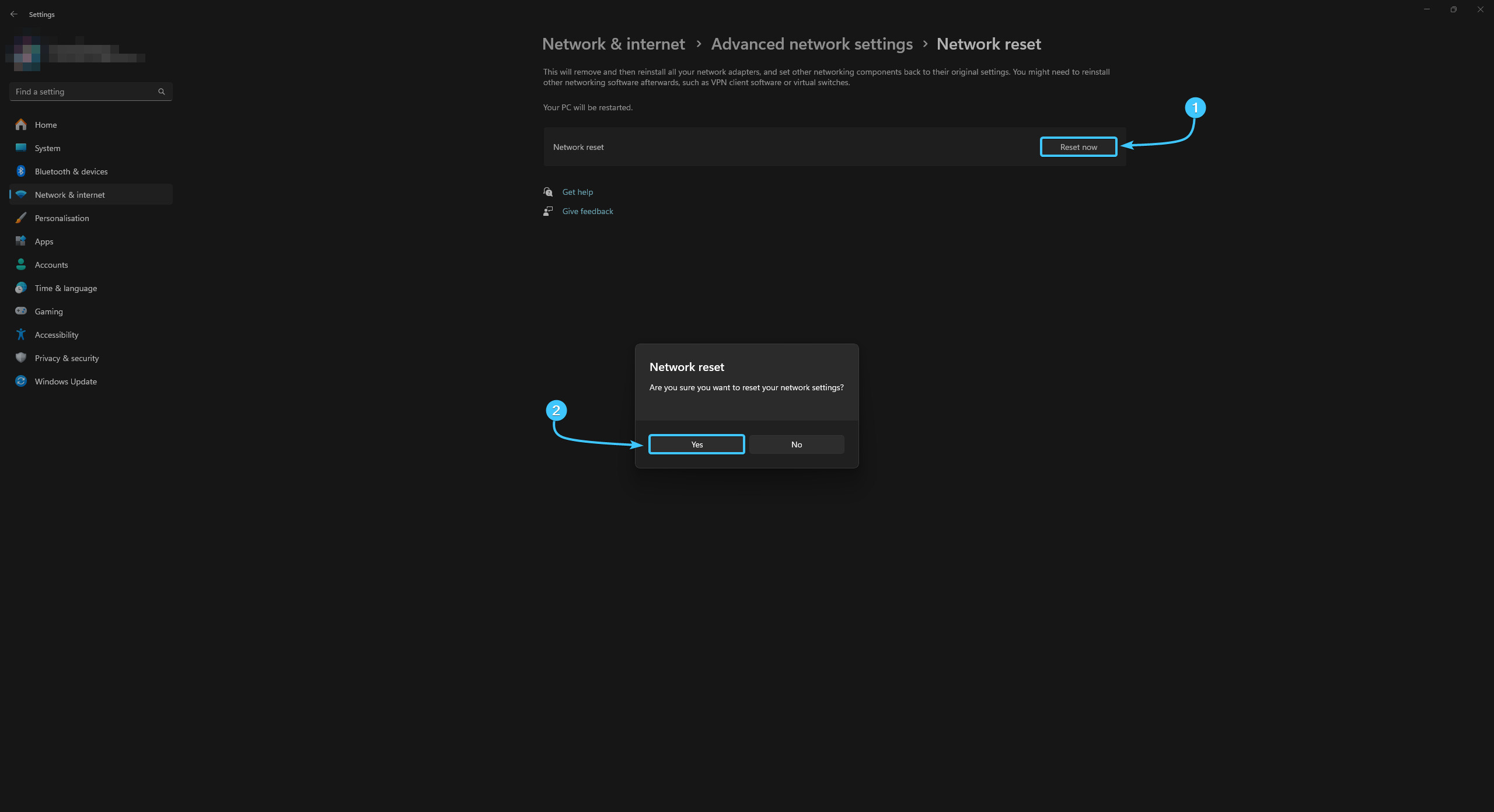The image displays a software interface with a plain white background, making legibility challenging despite attempts to zoom in. On the left side of the screen, there is a vertical menu consisting of multiple selectable items, each accompanied by an identifying icon to its left. At the top of this menu is a search bar or text box, above which lies a blurred section.

To the right of the screen, there are several headings and subheadings: "Network and Internet," "Advanced Network Settings," and "Network Reset." Beneath these headings, there is descriptive text, although the exact content is not specified. Additionally, there is a gray rectangular box containing text that is not properly described. Below this, there are two lines of text, each prefaced by distinct icons on the left.

A blue square with an arrow, featuring a circular end, points towards an element on the screen, indicating an area of interest or interaction. Further down, a pop-up window emerges with a title starting with "Network," offering Yes and No buttons for user input. The "Yes" button is highlighted with a blue outline, suggesting it is the current selection or recommended action.